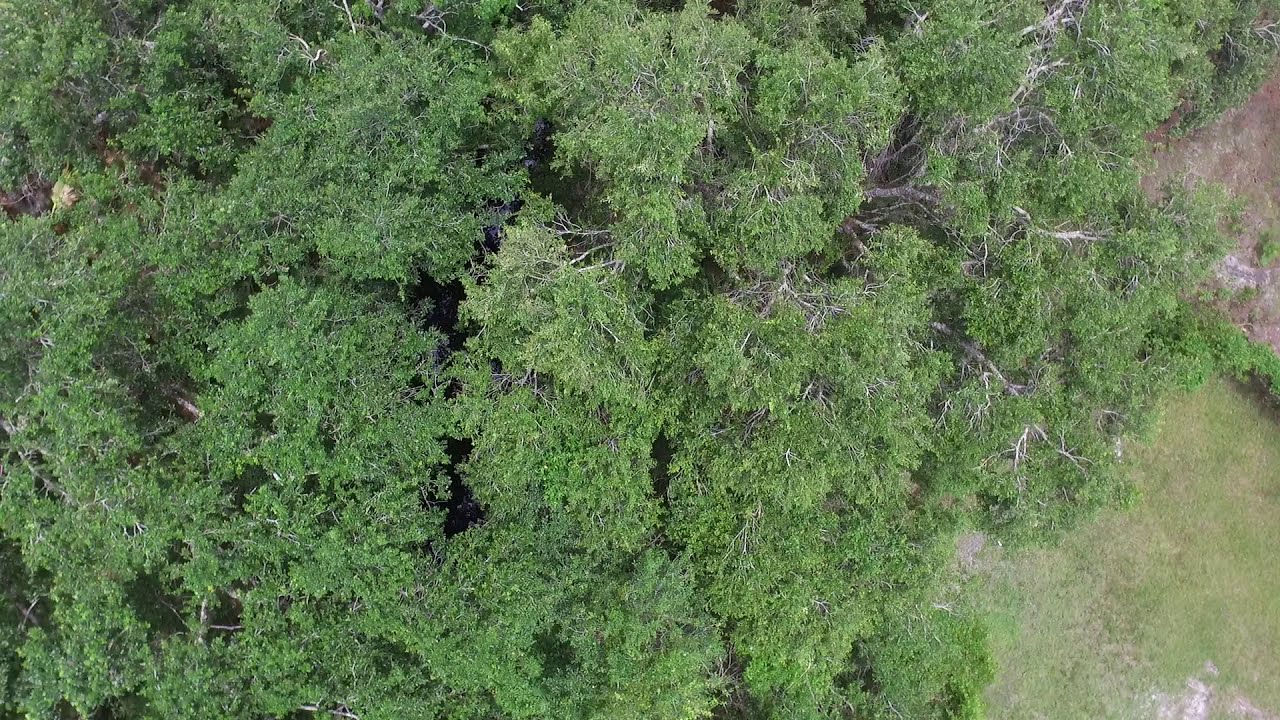The image captures an aerial view of a lush, green forest, likely photographed from a drone. About 80% of the scene is dominated by the dense canopy of dark green leaves and white-barked branches of the trees, suggesting a vibrant spring or summer season. The foliage, a mix of light green and dark green leaves, covers almost the entire frame. On the bottom right corner, there's a noticeable patch of thin grass interspersed with patches of brown soil, rocks, and possibly a part of a hill or cliff with reddish rocks. The left side of the image is densely packed with treetops and intertwining white branches. The photograph provides a serene overhead perspective, highlighting the rich greenery and subtle natural details of the forest landscape.